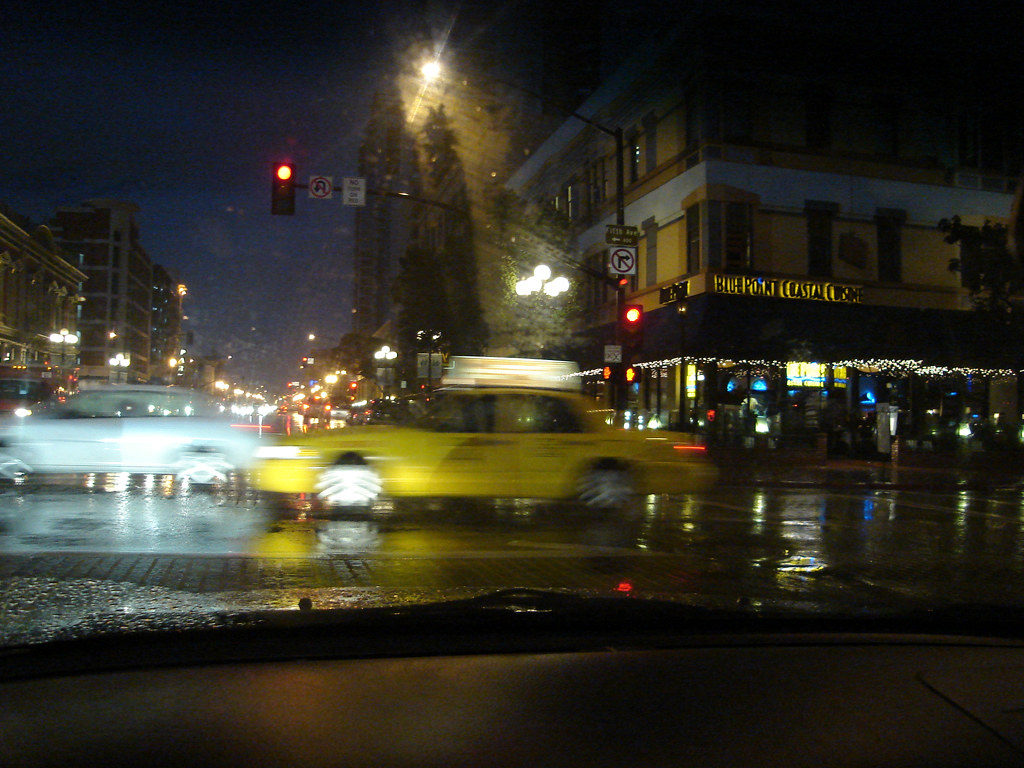A nighttime cityscape is captured from inside a car, with the vehicle’s body and windshield wipers visible at the bottom of the frame. The bustling street ahead features a lively scene with several cars zooming past from right to left, their motion evident through blurred trails. A distinctive yellow American taxi with a prominent sign on its roof speeds by, while a white sedan is also seen in motion on the far left, illuminated by streetlights. In the backdrop, a traffic light glows red, signaling vehicles to stop. The city’s buildings, adorned with decorative lights, add a charming glow to the scene, further brightened by numerous streetlights and the headlights of passing cars.